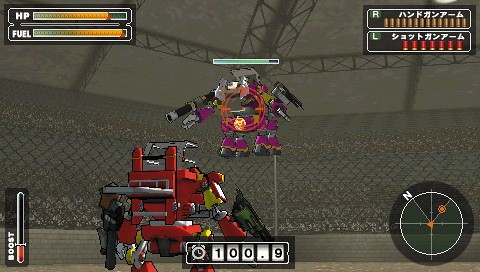The screenshot from the video game captures a dynamic scene set in a gray, dome-like stadium with visible truss work. At the center of the image, a purple and orange mecha suit, with a round body and four projecting limbs, appears to be midair with its gray hair-like feature adding to its alien aesthetic. The foreground shows the back of a red robot suit, equipped with guns in both of its extended, white arms, aiming downward. Various game interface elements are displayed: in the top left, an HP bar and a fuel bar; in the top right, ammo indicators with R and L labels and lines; in the bottom left, a boost bar with a small red segment; and at the bottom center, an old-style clock reading “100.9”. Additionally, the lower right corner features a compass within a black circle, with the N direction angled to the left. The overall pixelated, 90s-style graphics add a nostalgic charm to the combat-focused scene.